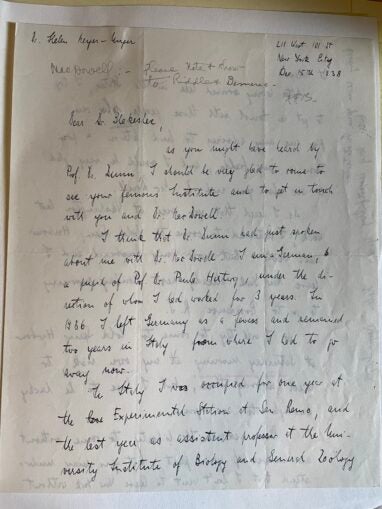This image captures a photograph of a delicate letter on a translucent, possibly rice paper, sheet, under professional studio lighting. The paper shows visible indentations from prior folding. Written in cursive ink, likely with an ink quill, the letter occupies the entirety of the page, suggesting it was composed on both sides, as faint writing is visible through the thin material under the light. 

On the top right, there's a date, "December 15th," and an address, "West 101 Street, New York City." At the top left, there is a faint "number one." The letter appears formal, beginning with a salutation, such as "Dear," directed to an unspecified recipient. It continues into several paragraphs, hinting at the importance of the correspondence. One can discern cursive scripts and smudged ink marks, adding to the letter's vintage allure. The photograph details the intricate folds and highlighted edges of the paper, enhancing its antique essence and the meticulous nature of the handwriting.